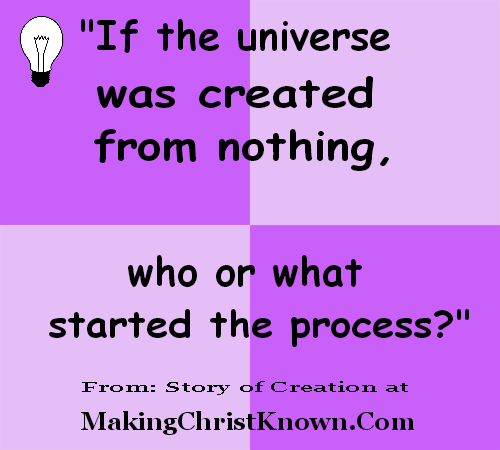The image is a single figure composed of four smaller squares forming a larger square, arranged in a grid pattern. The top left and bottom right squares are a dark lavender purple, while the top right and bottom left squares are a lighter lavender shade. In the top left square, there is an image of a light bulb. The figure also includes a text quote in black Comic Sans MS font that stretches over the top two squares and continues over the bottom two squares. The quote reads, "If the universe was created from nothing, who or what started the process?" Below this quote, another line of text reads, "From: story of creation at makingchristknown.com," in a more standard font. The overall design resembles a slide from a slideshow, possibly intended as an advertisement for church services.